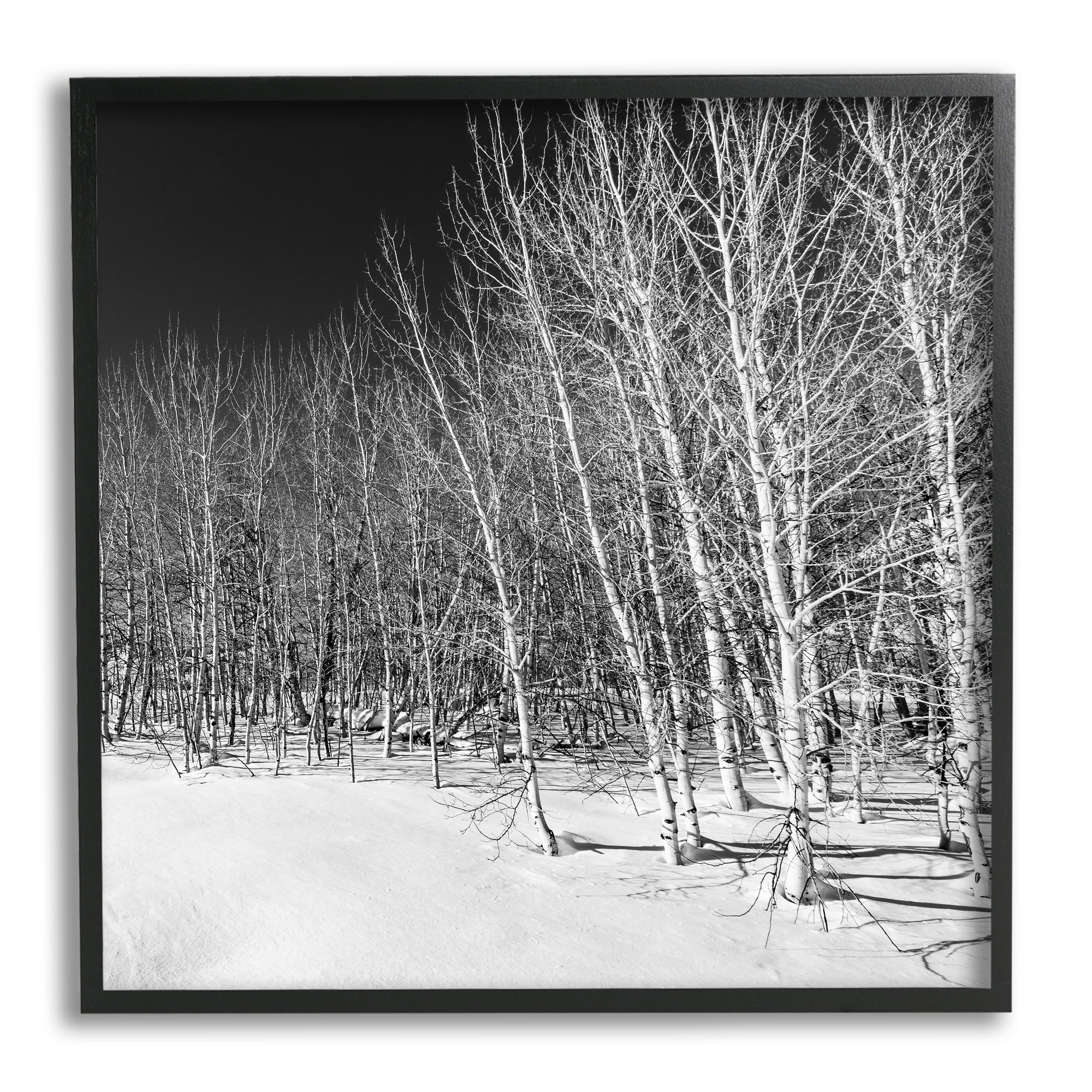This is a square-framed image, possibly a drawing or photograph, depicting a serene winter landscape predominantly in black, white, and various shades of gray. The thin, black frame encloses a snow-covered ground with a line of leafless birch trees positioned centrally, their white trunks speckled with black spots. The branches, also white and devoid of leaves, extend in various directions. In the background, the sky transitions from dark grey to black, focusing this dark gradient in the top left corner of the image. The overall setting is nighttime, further emphasized by the deep, dark sky, enhancing the stark, wintry atmosphere of the scene.